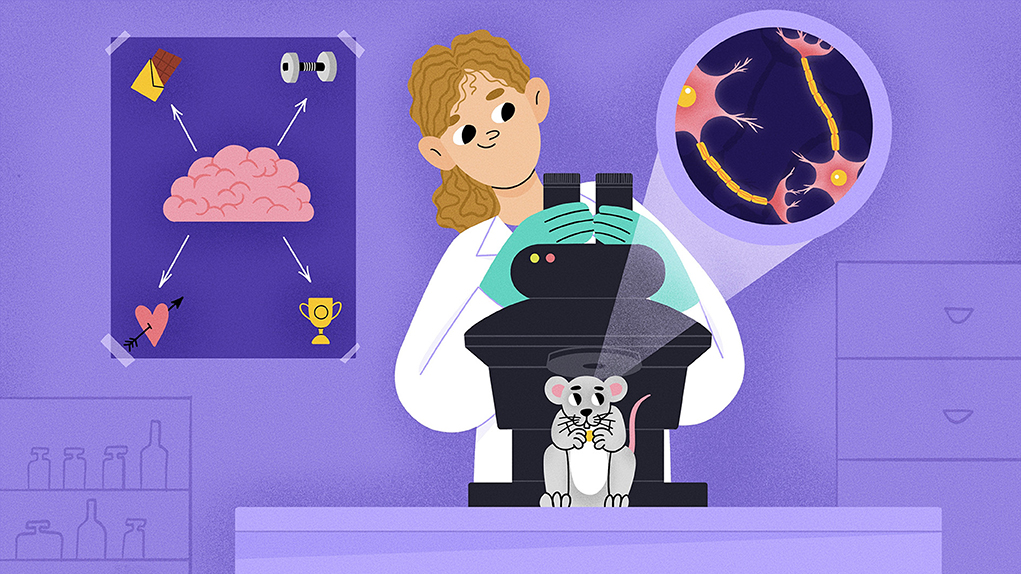This color illustration, set in a landscape orientation, features a cartoon depiction of a woman scientist in a laboratory, deeply engaged in her work. She is wearing green gloves and is focused on a black microscope. Underneath the microscope, a mouse is seen nibbling on a piece of cheese, seemingly unperturbed. In the top right corner of the image, there is a magnified view, presumably from the microscope, showing a detailed neurological illustration of a mouse's brain with pink membranes and yellow structures. The mouse appears anxious, glancing up at this enlargement.

In the background, the laboratory setting is accentuated with a dark purple cover. On the top left corner, a prominent poster showcases a pink brain with arrows pointing towards illustrations symbolizing various capabilities of the brain such as weightlifting, trophies, hearts, muscle, creativity, and chocolate. The overall style of the illustration is vibrant and detailed, capturing the essence of a scientist's world of discovery and ingenuity.